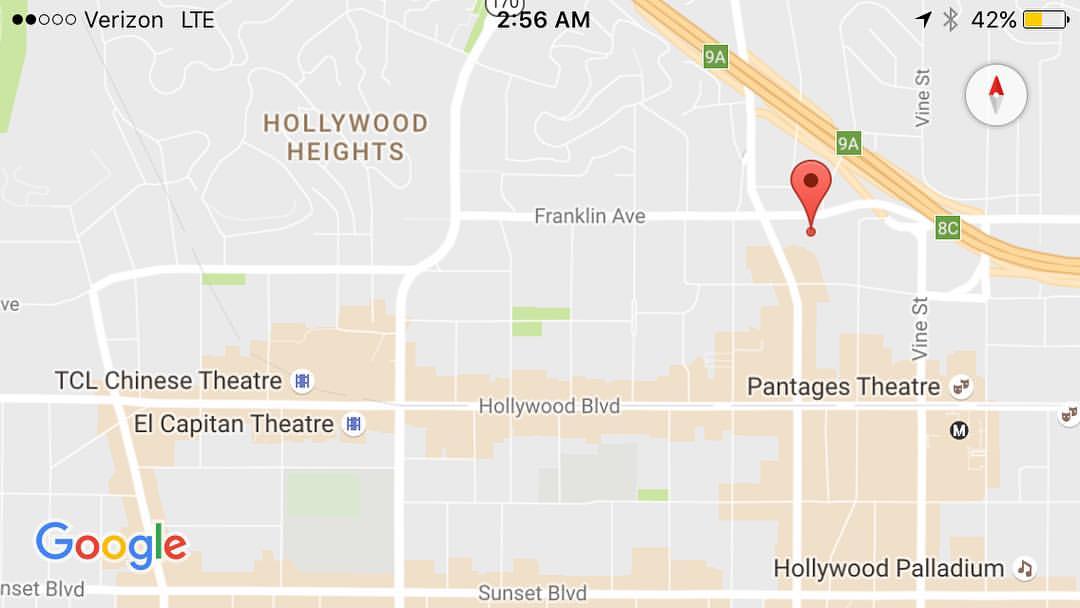This image is a detailed screenshot of Google Maps focusing on Hollywood Boulevard in Hollywood, California. Featured prominently on the map are several iconic landmarks. The TCL Chinese Theater is easily recognizable, marked as a significant point of interest. Directly across from the TCL Chinese Theater is the El Capitan Theatre, another renowned venue. Moving along Hollywood Boulevard, the Pantages Theatre is also noticeable. The map does not label the smaller streets and alleyways but highlights larger streets, including Sunset Boulevard to the south. Notably, on Sunset Boulevard towards the right, the Hollywood Palladium is visible. In the top left corner, the map designates an area as Hollywood Heights, indicating a residential neighborhood. The overall map showcases the significant cultural landmarks and historic theaters, reflective of Hollywood's storied history in the entertainment industry.